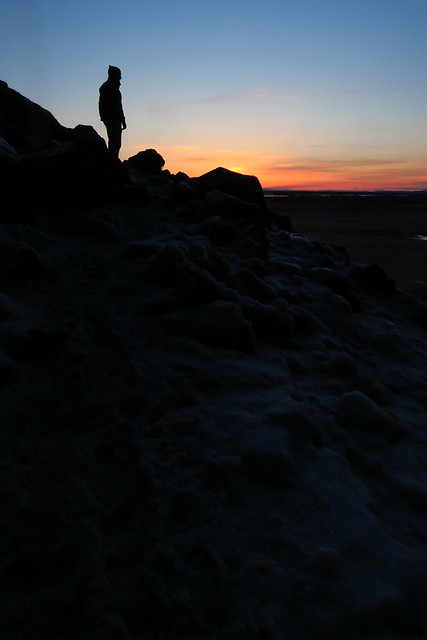A stunning photographic scene captures a lone man, clad in a hoodie, standing on a rocky incline during a sunset. The photograph, devoid of any text, focuses on the natural, serene beauty of the setting. The sun is just visible, protruding from behind a distant mountain, casting an orange and yellow glow across the horizon. Orange bands splice through scattered grayish clouds, with the sky transitioning to a deep blue at the top of the image. Most of the image, around two-thirds to three-quarters, consists of a dark, silhouetted foreground, accentuating the rocky outcrop on which the man stands. Positioned between two rocks, the man gazes towards the setting sun, his silhouette blending seamlessly into the shadowed landscape, imparting a sense of solitude and contemplation.